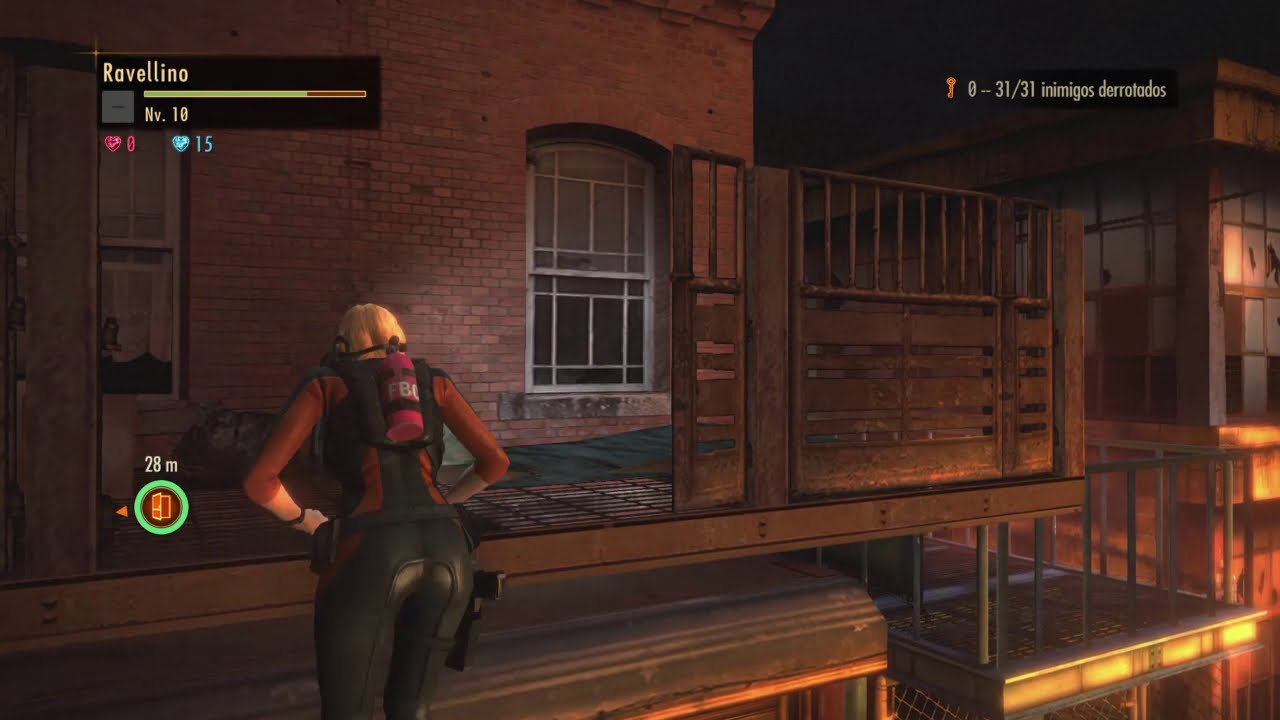The image is a screen grab from a third-person video game, featuring a blonde woman as the main character. She is outfitted in a red long-sleeved shirt, black pants, and a wetsuit with a red oxygen tank on her back. A gun is secured in a holster on her hip. The scene takes place at night and the lighting is dramatic, adding to the tension of the setting. The woman is in the process of pulling herself up onto a rickety, old iron balcony attached to a red brick building. Additional details include a name and health status bar in the upper left corner, an objective icon with distance indicators on the left side, and mission status text on the top right. The building is surrounded by elevated platforms and the brick wall is illuminated, possibly by a flashlight the character is holding.